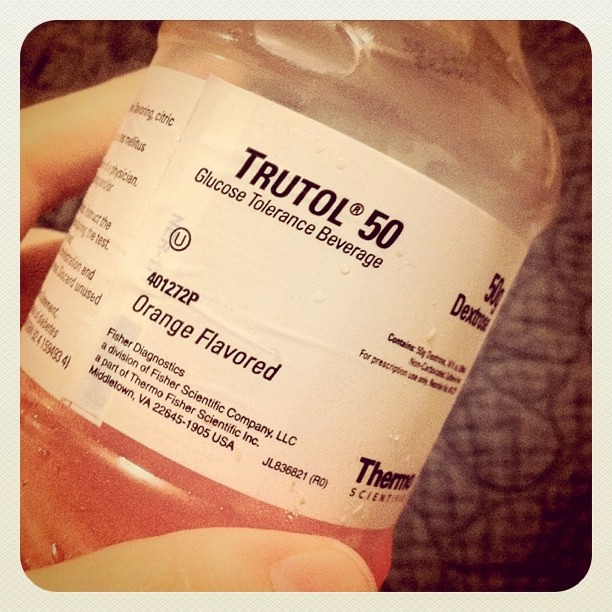A small, glass bottle is prominently featured in a close-up, Polaroid-style image. The bottle, tilted steeply from lower left to upper right, is held by a Caucasian person's hand, with the thumb gripping the front and several fingers supporting from behind. The focus is on a white label with dark text that reads "TrueTol 50," identifying the bottle as a glucose tolerance beverage. Near the top right of the label, there is a lot code number, and below, in italicized letters, the flavor is noted as "Orange Flavored." The product was manufactured by Fisher Diagnostics in Middleton, Virginia. The bottle, used for glucose tolerance testing in diabetic patients, is partially full, revealing an orange liquid beneath the label. The top portion of the bottle, which is clear, is cropped out of the image.